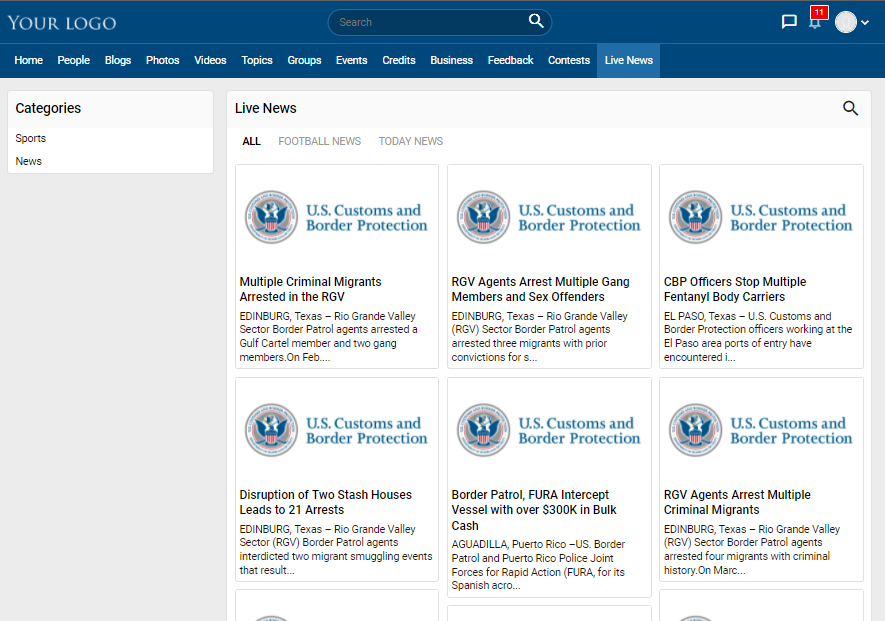The image is a screen capture from a desktop computer displaying a web page from the U.S. Customs and Border Protection website. The upper left section of the screen features the U.S. Customs and Border Protection logo, which is white on a blue background.

Below this main logo, there is a white section containing six smaller square frames, each of which showcases the same U.S. Customs and Border Protection logo. Each frame includes a paragraph of information related to recent activities or updates from the agency.

In the first frame located at the top left, the logo is positioned above a news headline written in black text. The headline reads: "Multiple criminal migrants arrested in the RVG," followed by a more detailed description: "Edinburgh, Texas, Rio Grande Valley Sector Border Patrol Agents arrested a Gulf Cartel member and two gang members on Feb."

The information highlights specific enforcement actions taken by border patrol agents in the Rio Grande Valley, emphasizing their ongoing efforts to combat criminal activities related to illegal migration.